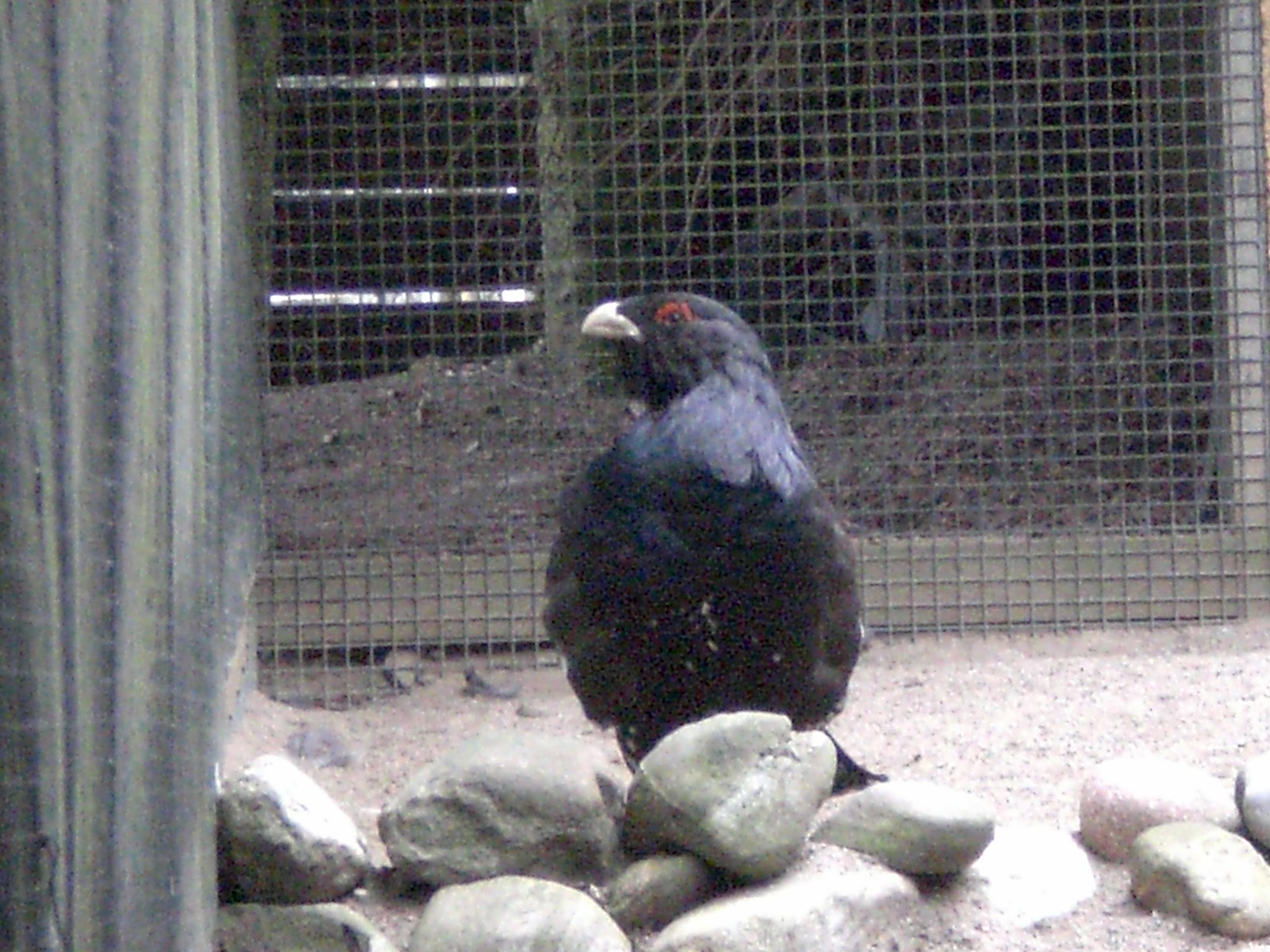In this photograph, we see a striking black bird situated inside a wired metal cage that resembles a chicken coop. The cage, with its fine cross-patterned wire mesh, is visible on the left side and in the background of the image. This enclosure appears to be part of a larger outdoor aviary or zoo exhibit, supported by wooden frames and possibly adjoining another animal pen, as evidenced by the suggestive background structures and distant foliage.

The bird stands on a base of white, fine-graveled arid dirt, mingled with scattered, rounded grey rocks. Positioned among these rocks, the bird displays a predominantly black plumage, merging shades of black, brown, and a hint of bluish hues, with its head turned slightly to the left, showcasing its distinct facial features. Above its black eyes is a prominent red eyelid or "eyebrow," while its short, curved beak appears white or whitish-yellow. This contrasting facial coloring is especially vivid against the bluish-white area on its neck and the purply-black tones of its body.

The background reveals hints of greenery and possible foliage, adding an element of natural habitat to the otherwise artificial enclosure. The image, although slightly fuzzy, captures the intricate details and unique attributes of this impressive bird, which, while it may bear a superficial resemblance to an eagle, is clearly a different species altogether.